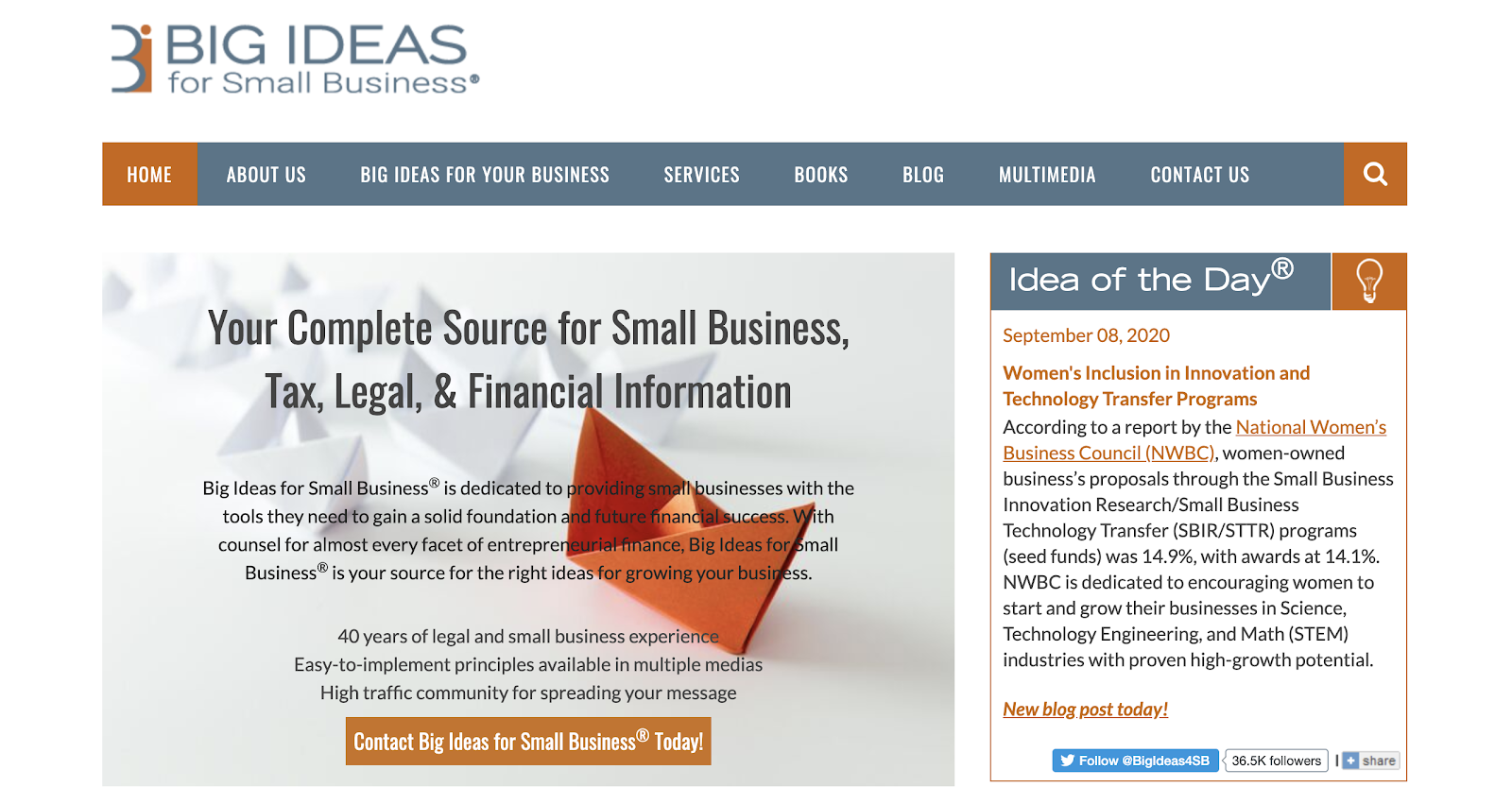Screenshot of the "Big Ideas for Small Business" website. The top navigation menu includes options such as Home, About Us, Big Ideas for Your Business, Services, Books, Blog, Multimedia, Contact Us, and Idea of the Day. The website's tagline reads "Your Complete Source for Small Business, Tax, Legal, and Financial Information." The design features a white background with a gray top section and orange search buttons. A call-to-action invites users to contact Big Ideas for Small Businesses today.